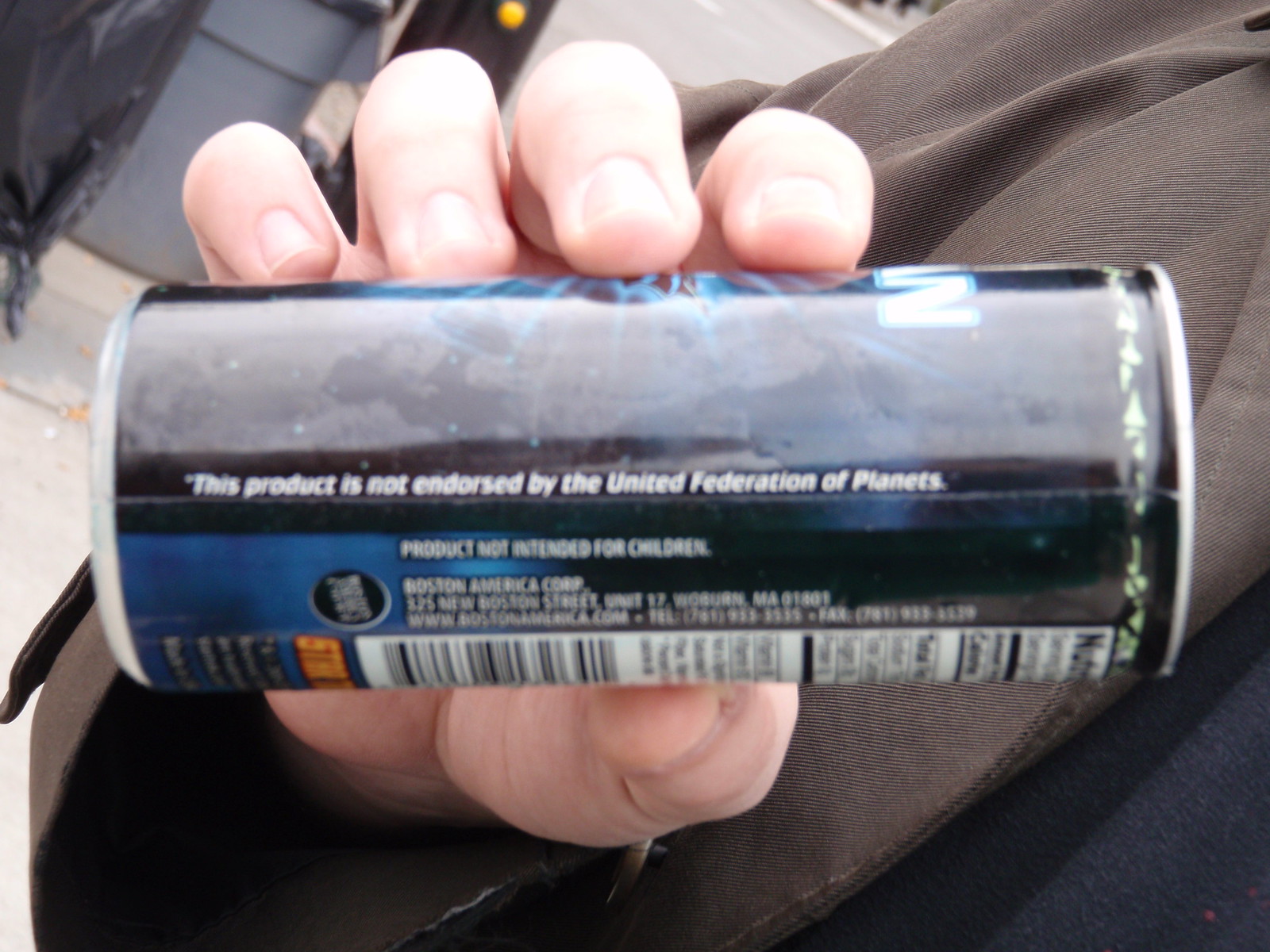In this image, a close-up captures a light-skinned person's hand holding a slim energy drink can, positioned sideways, while standing outside on a light gray sidewalk. The person is dressed in a dark brown jacket over a dark blue undershirt. To the left, a gray trash can with a black trash bag is visible, alongside another black trash bag. The can, predominantly blue and black with silver rims, displays white text, including "this product is not endorsed by the United Federation of Planets" and "product not intended for children." The manufacturer information, though slightly blurred, mentions Boston America Corp at "325 New Boston Street, MA 01801" with contact details and a website. A small green-rimmed pattern accents the can. The lid of the can is silver.